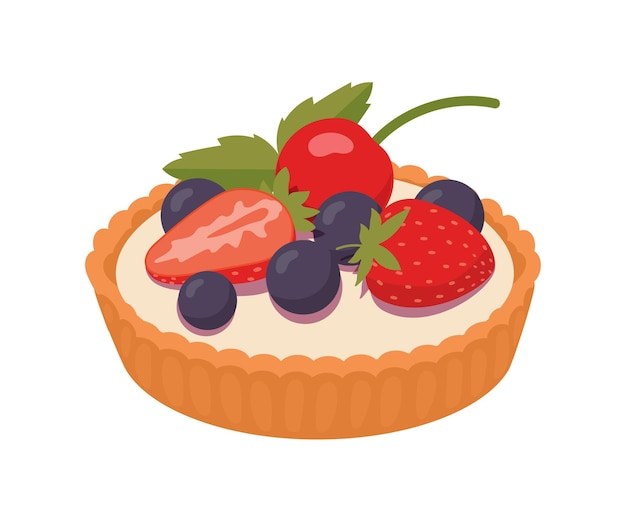A cartoonish image of a fruit tart is displayed from an isometric 30-degree angle. The tart features a scalloped, golden-brown crust encasing a creamy white filling, possibly vanilla pudding. Atop the filling, a variety of colorful fruits and garnishes are arranged. Among them is a whole strawberry with its green top still attached, a half-cut strawberry showing its inner part, and a large, vibrant cherry with a green stem and two small leaves. Complementing these are five blueberries of varying sizes and what appear to be sprigs of mint. Collectively, these elements contribute to the tart’s playful and appealing appearance.